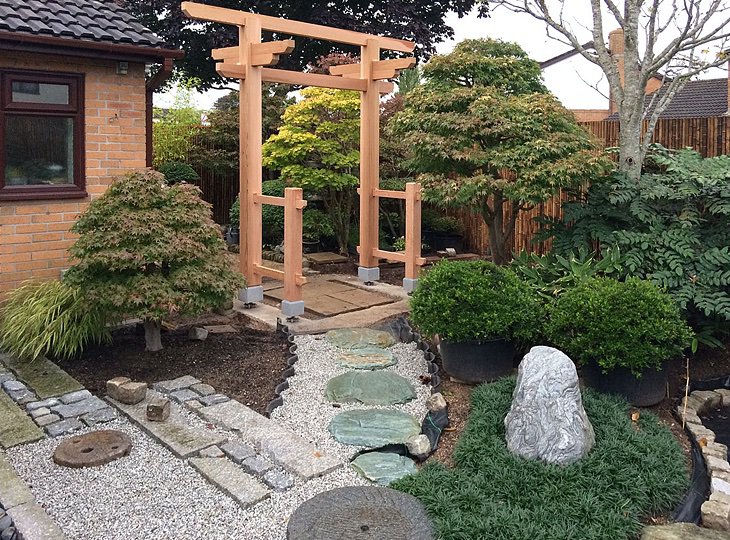This is an image of what appears to be an Asian-inspired, ornamental garden, situated in a backyard or possibly behind a business. The garden is set against the backdrop of a brick building with a black tile roof, though only the corner of this structure is visible. Central to the scene is a light wooden trellis or pergola, framed by various lush plants and trees including fern-like bushes and a bonsai-style tree. The garden pathway, featuring a combination of turquoise teal stepping stones and smaller pebbles, seems to be a work in progress, adding an unfinished yet serene aesthetic. A wooden fence in the background partially conceals another house, indicating a residential setting. The vivid greenery, diverse mix of materials, and intricate landscaping elements create a striking and tranquil environment.